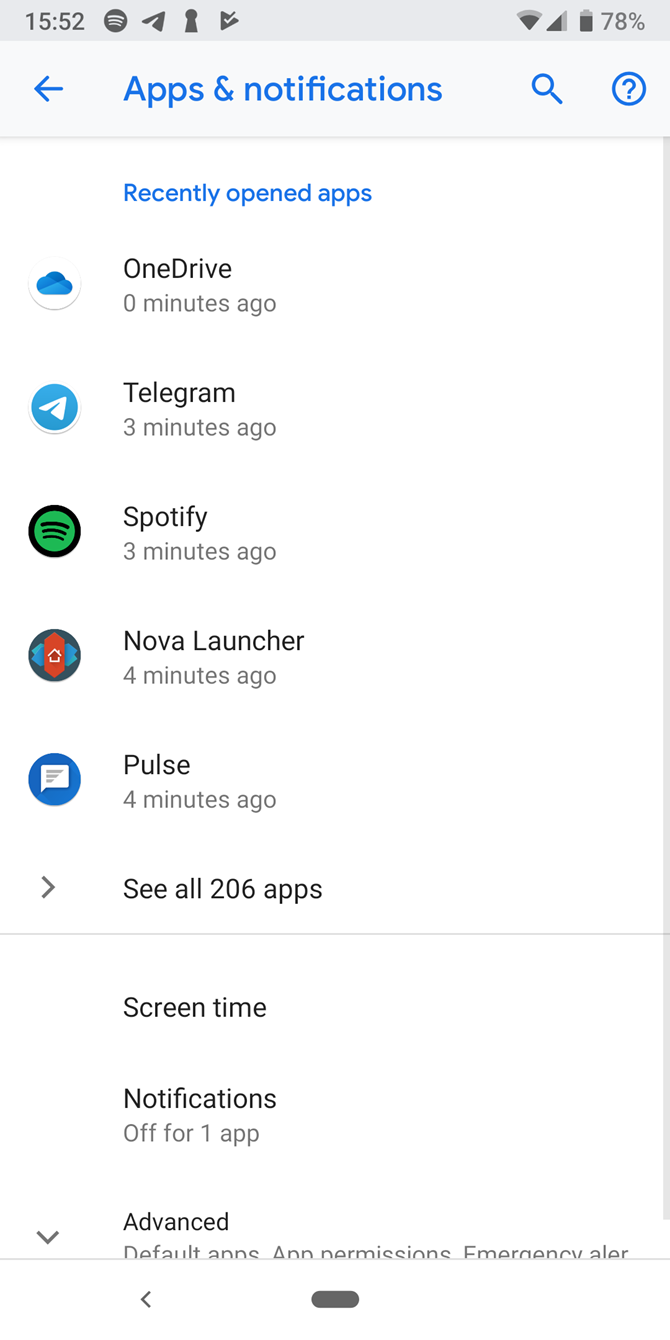The image depicts a smartphone screen showcasing recent app activity and notifications. At the forefront, the "Recently Opened Apps" section is highlighted in blue. This section lists apps like OneDrive, accessed zero minutes ago; Telegram and Spotify, both accessed three minutes ago; and Nova Launcher and Pulse, each accessed four minutes ago. Below this, there's a "See All 206 Apps" option, indicating a lengthy list of other available apps. A gray separator lies beneath, followed by the "Screen Time" section. This section includes options for notifications and advanced settings.

At the top of the screen, several status icons are visible. These include indicators for broadband strength, the current time (15:52), and battery status, which shows 78% remaining. Additional icons visible include a lock, an airplane mode icon, and a triangle with a checkmark, amongst others.